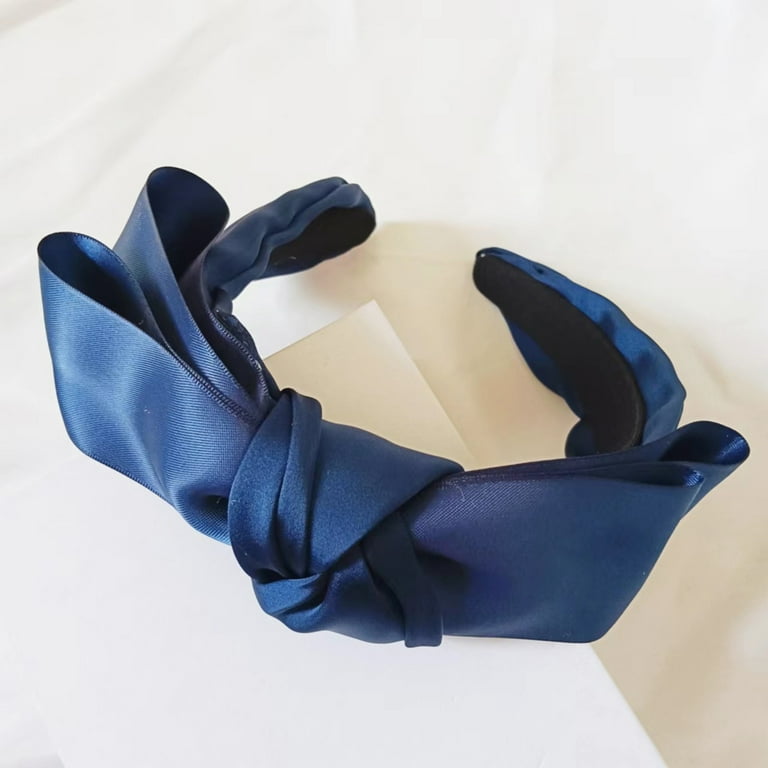The image depicts a silk or satin hairband positioned diagonally in the middle of a white surface. The hairband is primarily navy blue with a black fabric inner lining. Its distinctive feature is a decorative bow, tied at the top, presenting two prominent, draping flaps that create a bow-tie appearance. The headband is C-shaped and designed to clasp onto the head, suggesting it is a type commonly worn by females. The overall material of the hairband is shiny, giving it a sophisticated look.